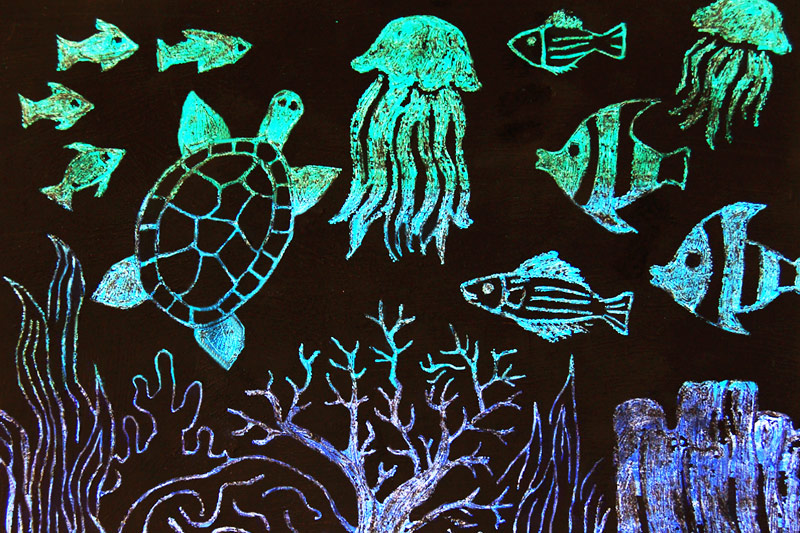The image presents a vividly detailed underwater scene, seemingly created on a black chalkboard with neon, glow-in-the-dark chalk. The landscape, slightly wider than it is tall, transitions in color from a teal at the top, through light blue in the middle, to purples at the bottom. Highlighted against this backdrop are various sea creatures and underwater vegetation. 

On the left, a small school of green fish swim to the right. Moving rightwards, a green and teal turtle swims upward towards approximately one o'clock. Adjacent to the turtle, a green jellyfish floats. Further to the right, another diverse school of fish, showcasing shades of green, black, and blue, swim to the left. In the upper right corner, another green jellyfish drifts.

Below these creatures, the seabed is bustling with vivid vegetation, including purple and teal sea plants, seaweed, and coral formations that span a range of blue and purple hues. These details culminate in a rich, colorful underwater tableau that vividly contrasts with the solid black background, showcasing the various shades and intricate designs characteristic of a scratchboard art piece.